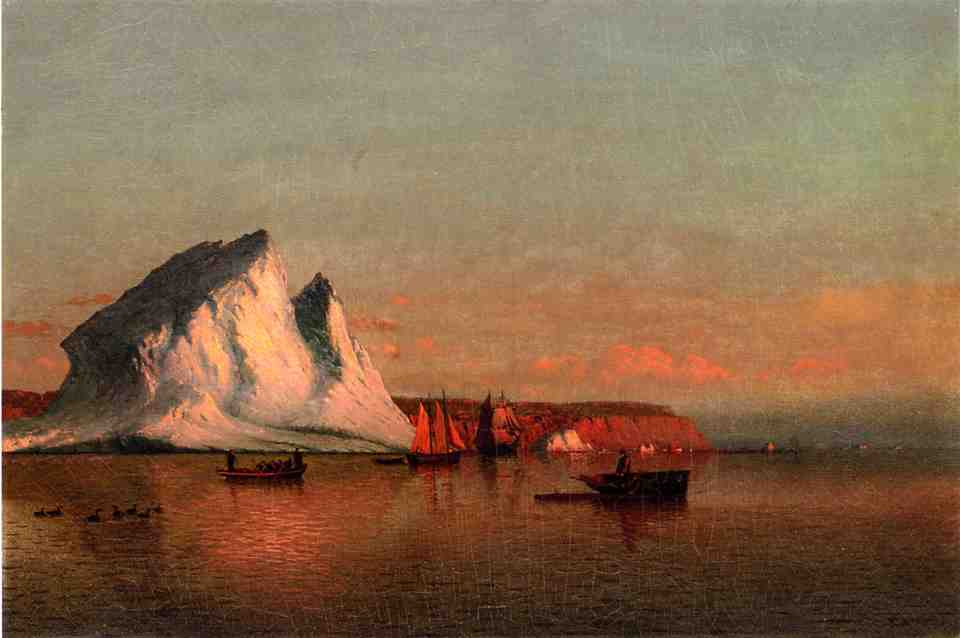A serene, oil-on-canvas masterpiece captures the tranquil scene of a vast, smooth sea bathed in the warm hues of a sunset. Amber-tinted clouds fill the sky, casting a reddish glow upon the water that stretches from one side of the canvas to the other. To the left, a towering, white glacier dominates the scene, its shadowed side darkened and its sunlit face glowing. At the base of the glacier, on the right, lies a patch of flat land, possibly grass-covered.

In the lower third of the painting, six ducks swim near the left side, adding a touch of life to the serene waters. Adjacent to them are two rowboats; one, filled with several people rowing, sits alongside another nearby boat with a person standing. In the distance, two sailboats approach the shore – one resembling a grand pirate ship with multiple sails, and another smaller sailboat.

The texture of the painting reveals signs of age, yet it vividly captures the calm and reflective nature of the scene, with cliffs reflecting the sun's glow along the water's edge as it stretches toward the horizon. The overall effect is a calming, almost otherworldly depiction of nature intertwined with human presence, all bathed in the warm light of dusk.